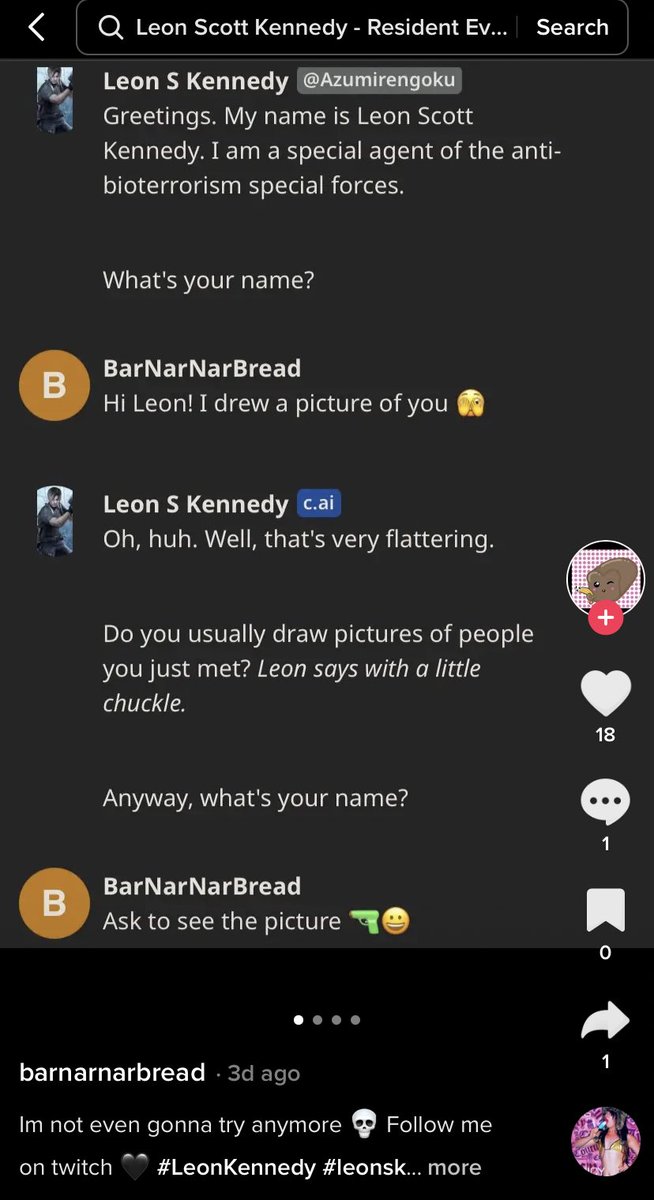Screenshot of a mobile app interface featuring a chat conversation:

At the top of the screen, there is a black bar with a white search field. Within this field, there is a magnifying glass icon followed by the text "Leon Scott Kennedy - Resident Evil... Search".

Below this, the chat interface displays a text conversation. The first message is from "Leon S. Kennedy at Azumarangoku," who writes: "Greetings, my name is Leon Scott Kennedy. I'm a special agent of anti-bio terrorism special forces. What's your name?"

In response, a user named "Banarnar Bread" writes: "Hi Leon, I drew a picture of you," followed by an emoji of a yellow smiley face covering its eyes.

Leon S. Kennedy replies: "Oh, that's very flattering. Do you usually draw pictures of people you just met?" The message is followed by a line in italics: "Leon says with a little chuckle. Anyway, what's your name?"

Banarnar Bread then writes: "Ask to see the picture," accompanied by a golden pistol icon and a smiley face emoji.

At the bottom of the screen, there are four white dots, indicating the presence of additional options or messages in the app.